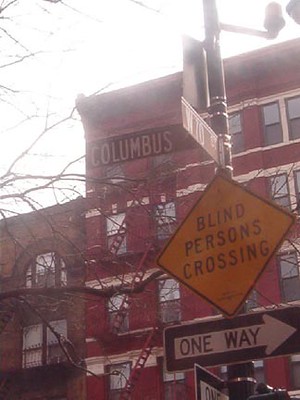The image depicts an urban streetscape dominated by a sizable brick building adorned with the name "Columbus." This structure, which appears to serve as an apartment building, features reddish brickwork and rises at least four stories high, with additional windows visible on a side wing. The facade is punctuated by numerous windows, suggesting a substantial number of units.

In the foreground, a yellow diamond-shaped sign warns of a "Blind Persons Crossing," while a black-and-white one-way street sign directs traffic. Both signs are partially obscured by a tree branch that intrudes into the frame, adding a natural element to the urban scene.

A small patio or set of stairwells with red ladders is visible on the upper levels of the Columbus building, hinting at external access routes or communal spaces for residents. Adjacent to this building is a smaller, brownish structure, also constructed with brick, contributing to the cohesive architectural aesthetic of the area.

The setting appears to be daytime under a somewhat foggy sky, casting a muted light over the scene. Additionally, there is a partially visible street sign that may indicate "W70," though the text is not entirely clear. Overall, the image captures the essence of a bustling city block with layered architectural elements and various public safety signs.